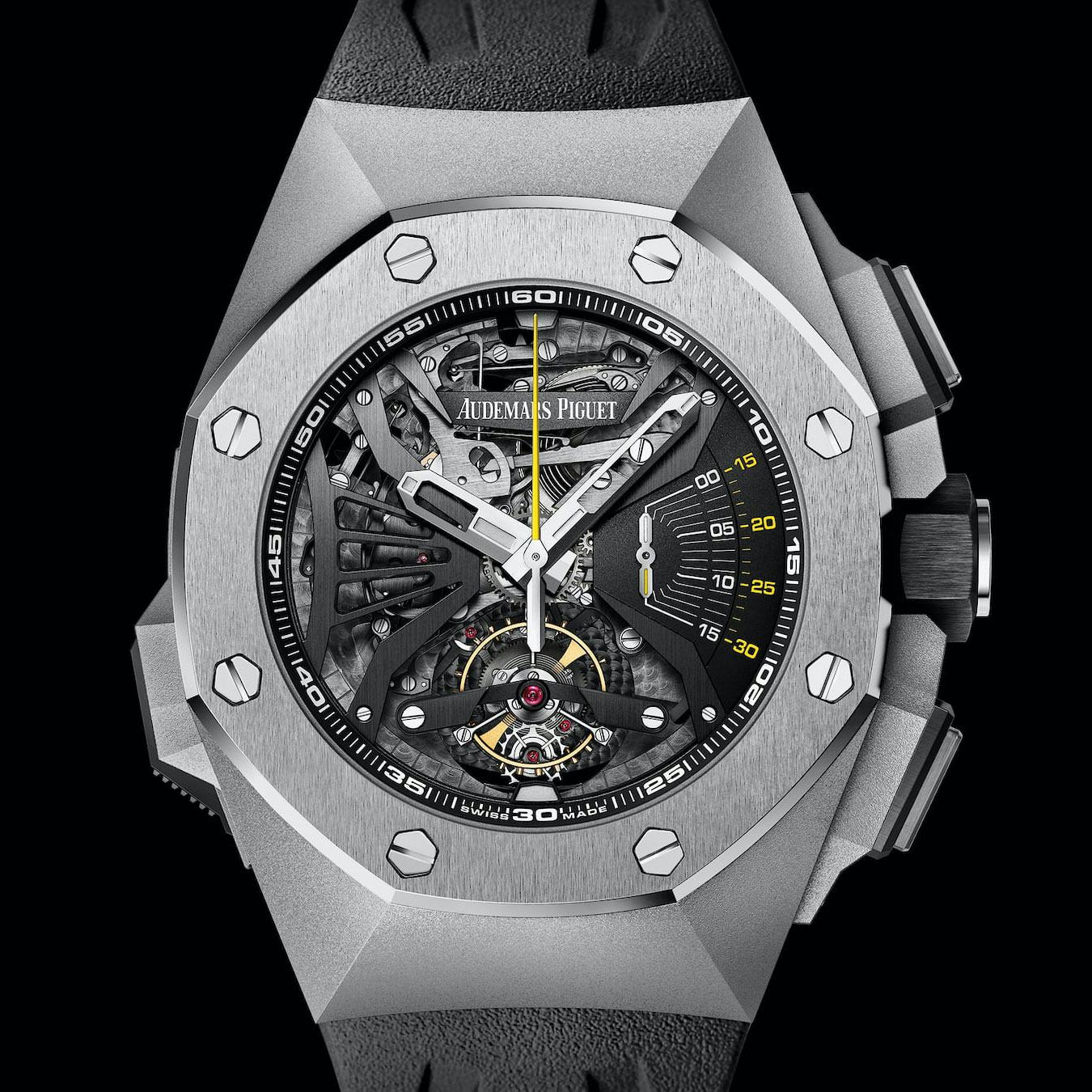This close-up marketing photograph showcases a sophisticated man's chronographic wristwatch from Audemars Piguet. The watch is encased in an octagonal, heavy, faceted silver metal case with eight rivets securing the rim to the case, which adds a robust allure. The photograph, set against a solid black background, highlights the intricate workings inside the silver-framed watch face. The dark gray interior reveals an array of visible mechanical gears, silver metal arms, and various chronographic gauges, all contributing to its high-tech, expensive appearance. 

The watch features a combination of hour, minute, and second hands; the hour and minute hands are metallic, while the second hand stands out in yellow. Numbers around the dial mark every 5-minute interval (0, 5, 10, 15, 20, 25, 30, etc.), and the right side includes markings for 15, 20, 25, and 30. There is a silver or stainless steel band partially visible; it may alternatively have black leather or plastic straps. The interior face is adorned with white hashtags and markings detailed at the top and lateral points on the watch. The piece includes three distinct buttons on the right side of the case: two silver and one black with a silver top, likely for adjusting the time and other functions. The name "Audemars Piguet" is inscribed on a lighter gray nameplate at the top center of the watch face, affirming its prestigious branding.